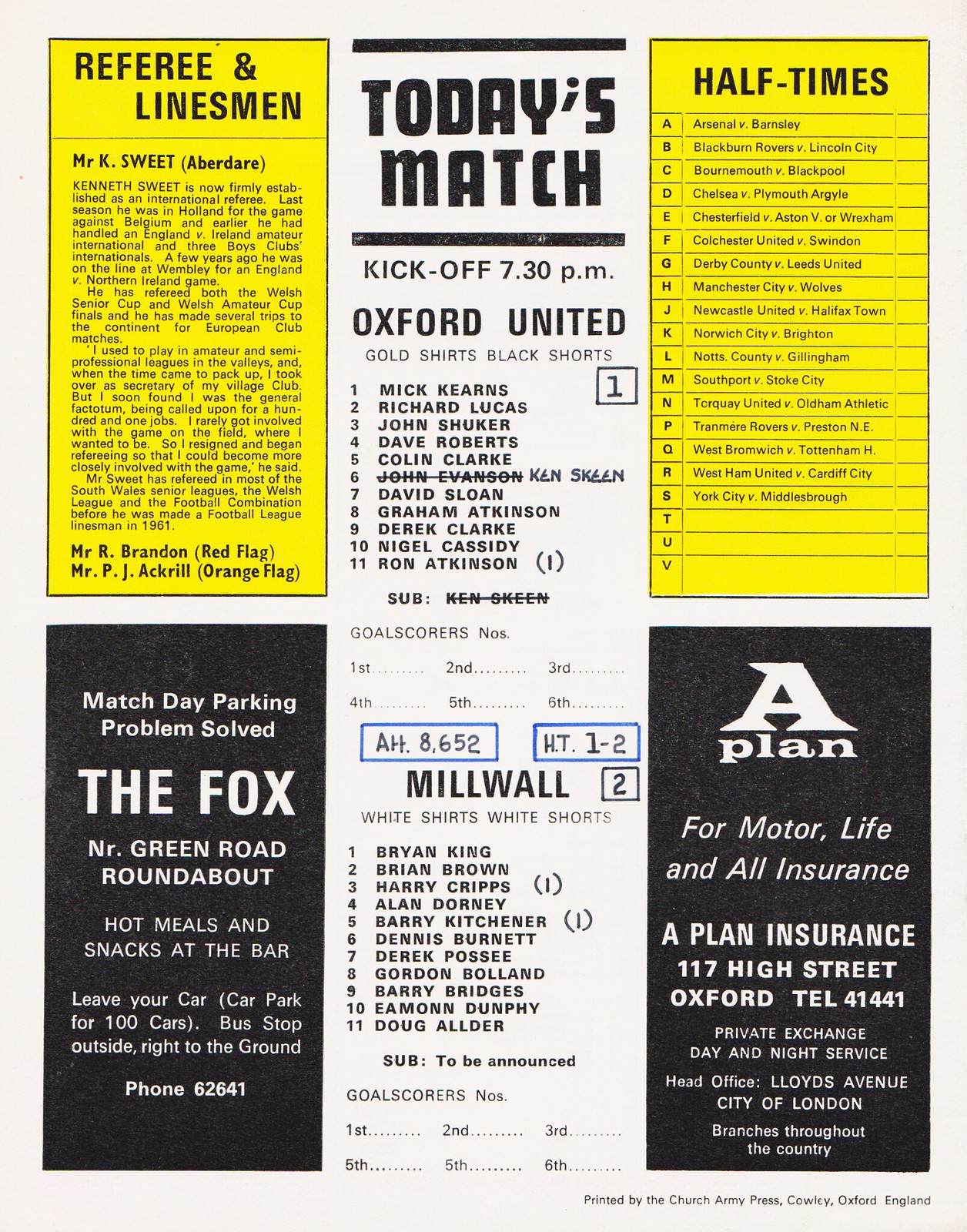This image is a scanned page from an older English football match day program, likely decades old, judging by its simple design and minimal colors. The page is divided into five distinct sections. The upper left corner features a yellow background titled "Referee and Linesman," listing the officials, including a detailed mention of Mr. K. Sweet. Opposite, in the upper right corner, another yellow section titled "Halftimes" lists scores from other matches such as Arsenal vs. Barnsley and Blackburn Rovers vs. Lincoln City. The center of the page, on a white background, prominently displays "Today's Match," Oxford United vs. Millwall, with a handwritten score indicating a 2-1 victory for Millwall. It also notes the kickoff time at 7.30 pm and lists the lineup for both teams, describing Oxford United in gold shirts and black shorts, and Millwall in white shirts and white shorts. The bottom left corner has a black rectangle ad for "Match Day Parking Problem Solved" at The Fox near Green Road Roundabout, mentioning amenities like hot meals, snacks, parking for 100 cars, and a bus stop to the ground. In the bottom right, another advertisement alerts readers to "A Plan for Motor Life and Oil Insurance" provided by A-Plan Insurance, located at 117 High Street, Oxford, with extended service details and branch locations across the country.